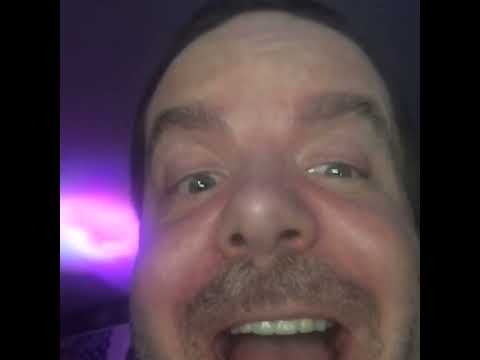The image captures a close-up of a middle-aged Caucasian man taking a selfie with a cheerful and surprised expression. His mouth is open, revealing a row of very white upper teeth. He sports a short, salt-and-pepper mustache and has short brown hair. His eyes, which appear to be a light green or hazel, are wide open, adding to his lively look. His cheeks have a slightly flushed color, possibly from blushing. The man has bushy eyebrows and a noticeable forehead. 

Behind him, the background features a vibrant purple light that casts a glowing effect across the area. This light, combined with the dim surroundings, gives the impression that the setting could be a nightclub or a similar venue. The wall behind him appears to have some form of decoration or wall art, although the details are obscured by the purple hue. The overall scene is dominated by this purple glow, contrasting with the dark ambiance surrounding the man's face.